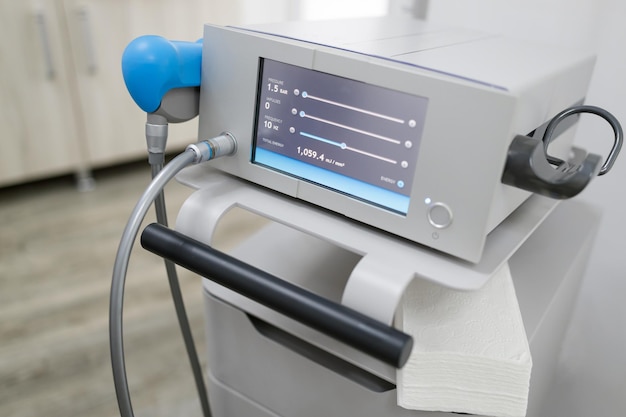The image features an indoor photograph of a beige, rectangular medical device prominently positioned from the lower right corner to the upper center-left area. The device, often seen in a doctor's office, sports a digital touch screen panel tilted slightly away from the viewer. The screen displays three horizontal lines of data, with the leftmost labels reading "1.5 bar," "0," and "10," and at the bottom, the text "Total Energy: 1059.4 millijoules per millimeter squared." Below the screen, black sliders allow for adjustments to pressure, impulses, and frequency. A dark gray cylindrical handle is visible near the device's lower section, with an additional hose connecting to a blue-capped component mounted on the left. In the right background, there's a blurred light-colored floor and a closed cabinet. Napkins can be seen placed in gaps within the machinery, adding to its clinical ambiance.